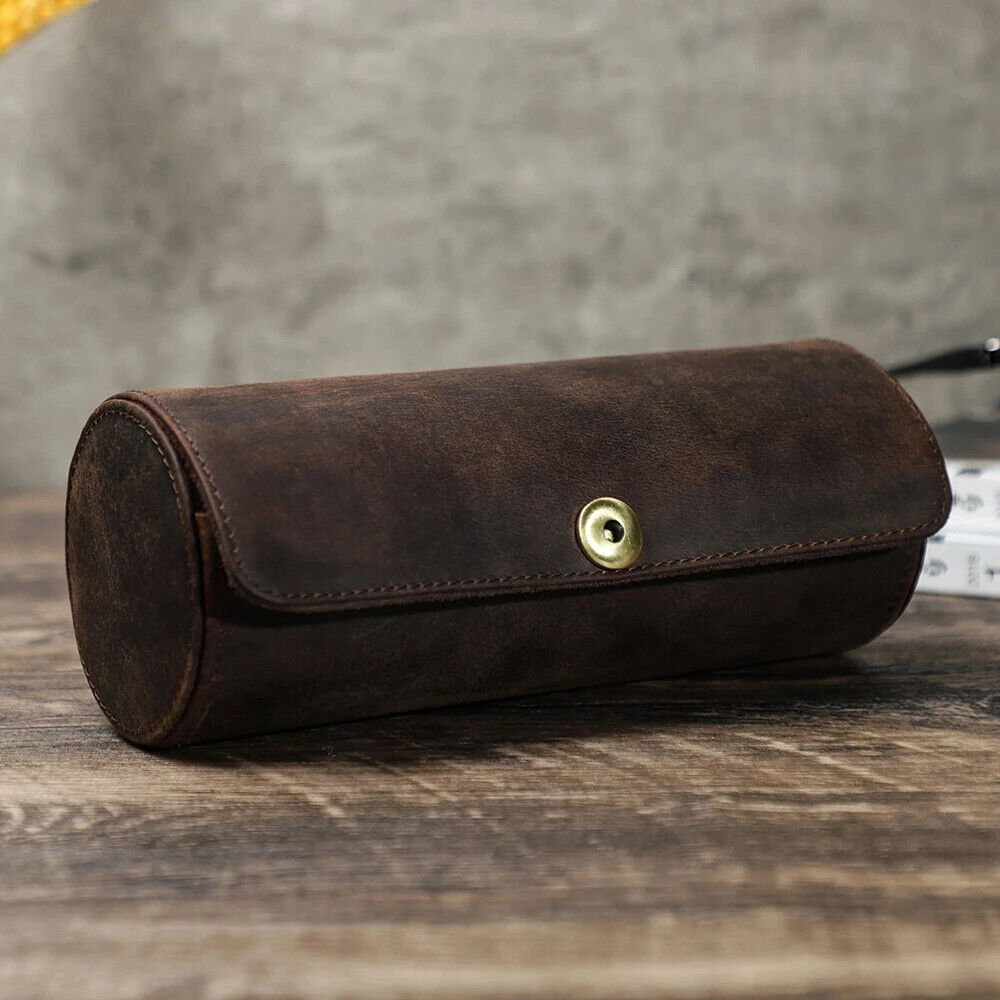This image features a cylindrical-shaped bag made of dark brown leather, prominently displayed on a weathered wooden table with varied light and dark brown striations and stains. The bag, potentially used as a purse or pencil case, lies at an angle from left to right. Its design includes detailed dark brown stitching along the edges and a distinctive flap closure, accentuated by a singular gold button at the center. The background reveals a white-grayish marbled wall, suggesting an indoor setting. Faint, blurred objects resembling boxes or books are discernible to the right, contributing to the image's depth and context.